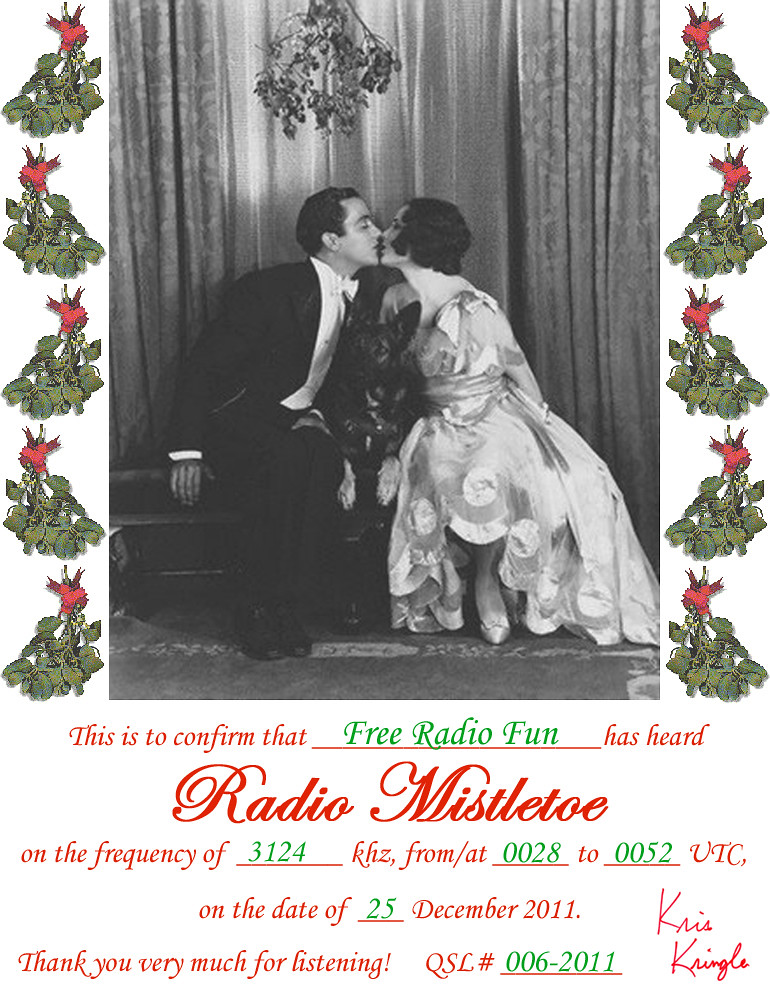The image is a black-and-white photograph from what appears to be the 1920s, featuring a newlywed couple kissing under mistletoe, with a German Shepherd between them. The man is dressed in a full tuxedo, and the woman is in a lavish white dress, characteristic of the era. The photograph is framed with Christmas-themed decorations, particularly mistletoe, on both the left and right sides. Below the image, there is text in red and green, formatted to confirm a radio signal reception: "This is to confirm that Free Radio Fund has heard Radio Mistletoe on the frequency of 3124 KHz from 0028 to 0052 UTC on the date of 25 December 2011. Thank you very much for listening. KSL number 0062011." The text fields for frequency and other specific details are filled in with green text. Finally, in the bottom right corner, the signature "Kris Kringle" appears in cursive writing, indicating the festive nature of the advertisement, which seems to promote a Christmas-time radio show.